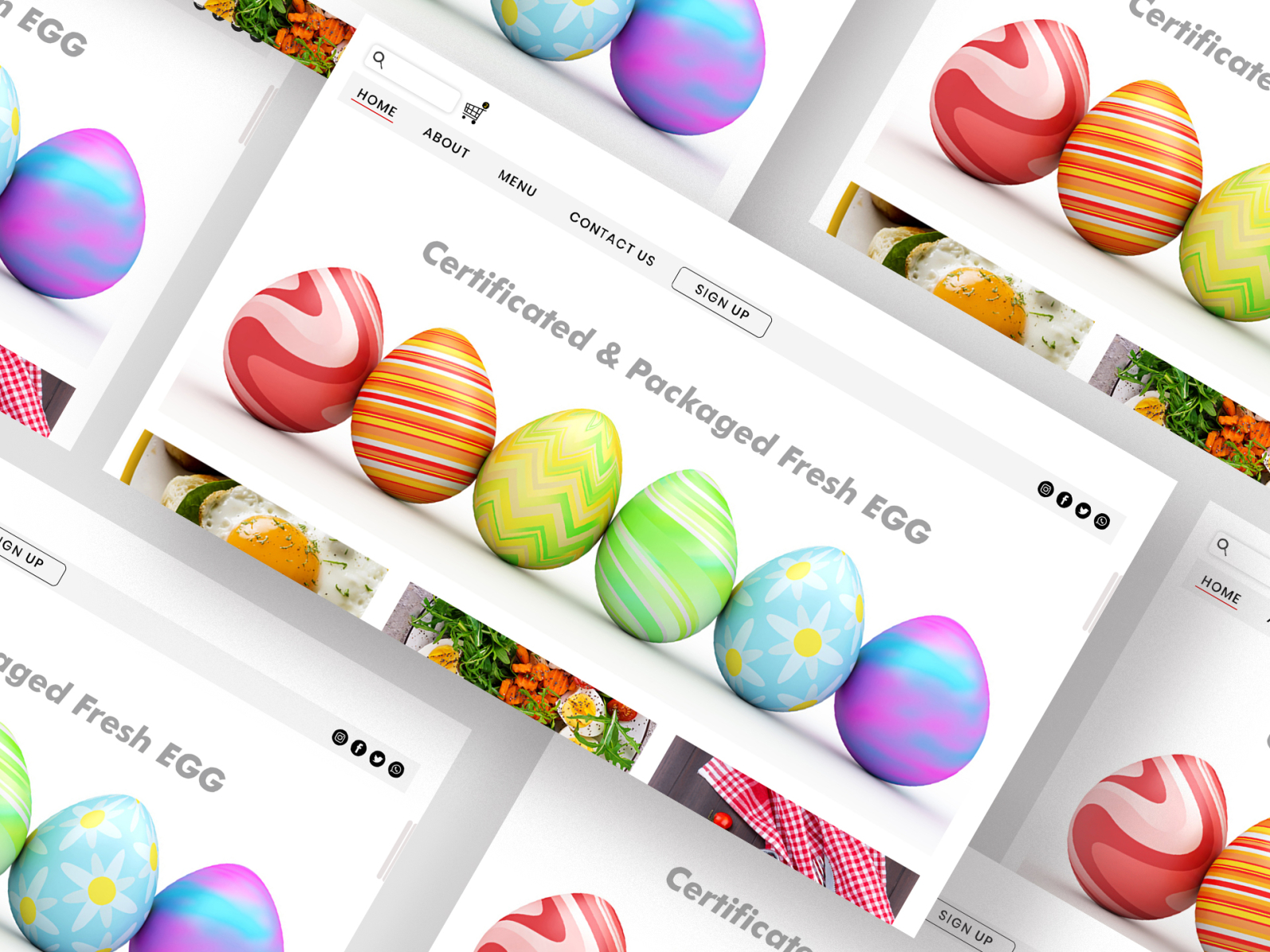The image depicts a webpage seemingly duplicated multiple times side-by-side to create a larger, continuous view. In the center of each webpage duplication is the primary image. At the top left corner, there's a search bar and a shopping cart icon, indicating that this is an e-commerce site. Directly beneath these elements, a vertical navigation bar lists several options: Home, About, Menu, Contact Us, and Sign Up. Adjacent to the navigation bar, on its right, are social media links, including Facebook, Twitter, and what appears to be Instagram, alongside an unidentified link.

The background of the webpage is plain white, providing a clean, minimalist appearance. Below the navigation bar, gray text reads, "Certified and Packaged Fresh Egg." 

Further down the webpage, there is a collection of six photographs showcasing elaborately decorated eggs. Five of these eggs are adorned with distinctive geometric patterns, while the fifth egg features a baby blue hue with delicate daisy decorations. 

It appears that there might be additional images beneath these photographs, likely demonstrating different recipes that utilize the eggs, but these images are partially cut off in the view. The entire scene of the webpage is repeated across the image multiple times, each iteration aligned seamlessly side-by-side.